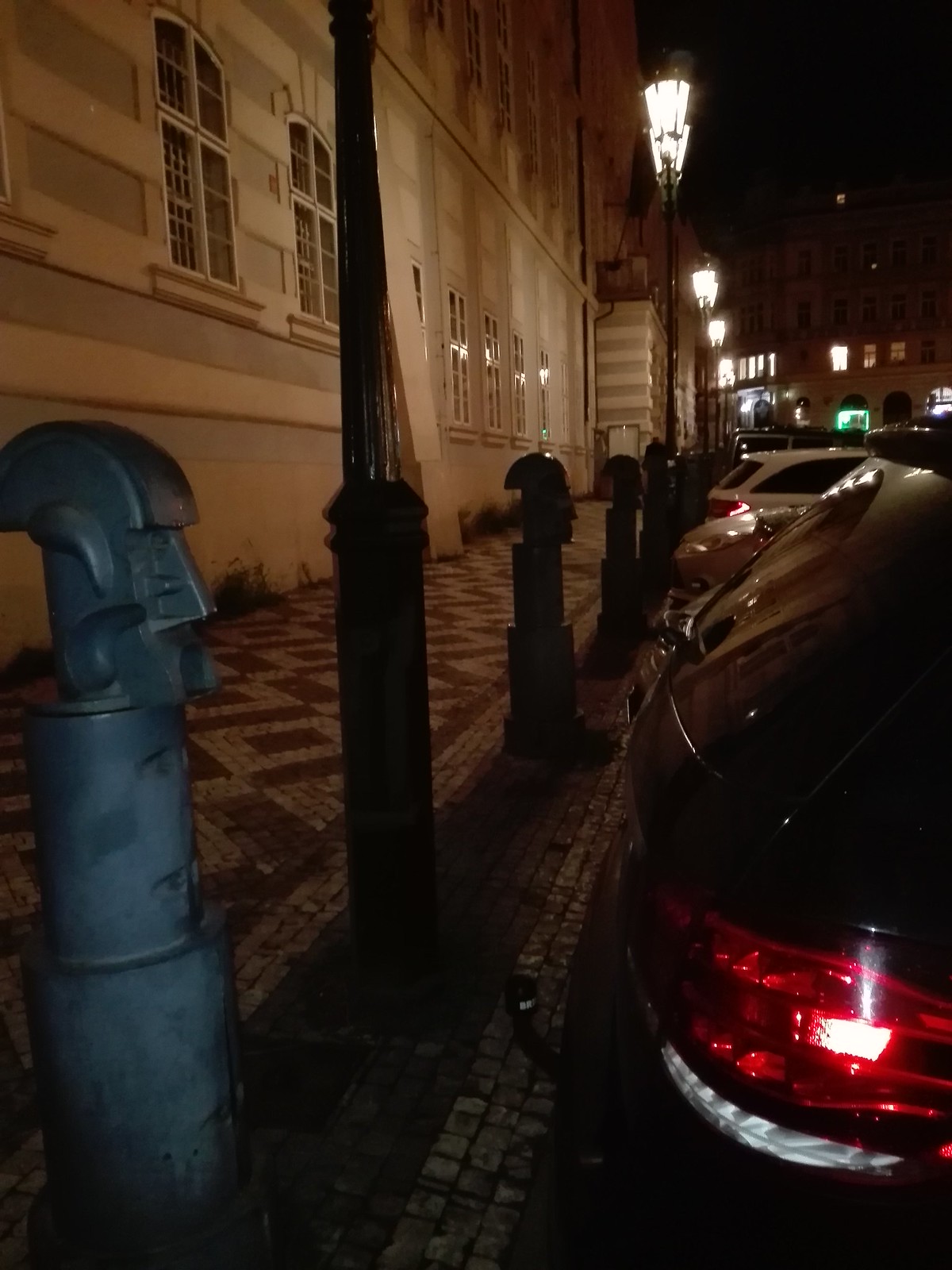In a nighttime city scene reminiscent of an old European city, several cars are parked along the curb, their taillights glowing in the dim light. A row of blue, metal parking meters, standing about four and a half feet tall, lines the sidewalk, which stretches from the foreground deep into the background, adorned with a red and white mosaic tile design in a geometric diamond pattern. The street is illuminated by ornate black iron lampposts, casting a warm light on the scene. To the left, a large, imposing building with green and white hues and large windows dominates the landscape, adding to the vintage atmosphere. Further down the street, additional buildings with lights in their windows and more vehicles can be seen, completing this striking and atmospheric cityscape.